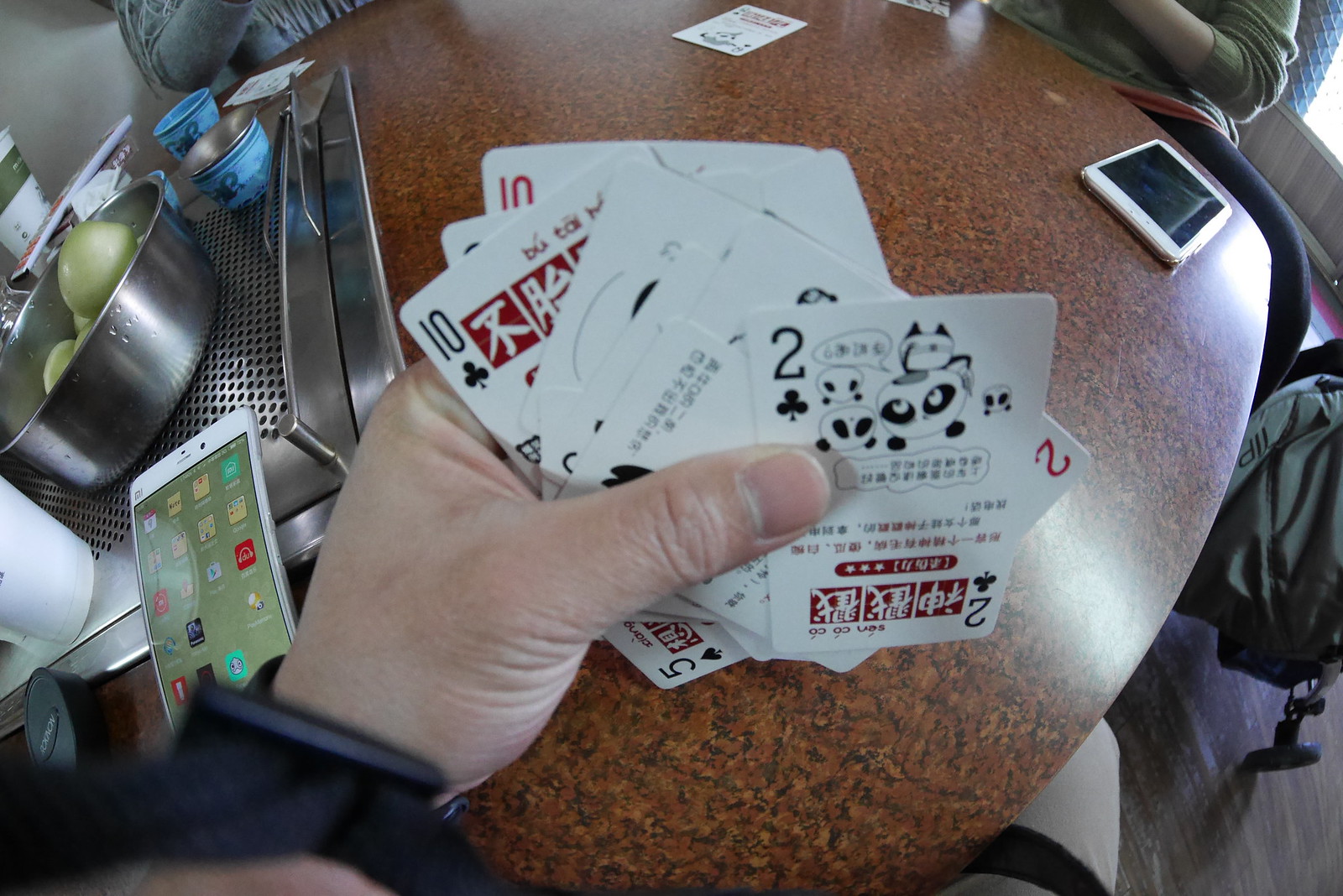A close-up photograph features a hand holding a fan of playing cards adorned with numbers in the corners and distinctive symbols of clubs, hearts, and spades. Each card is marked with unfamiliar Asian script, potentially Japanese, Chinese, or Korean. The hand holding the cards is the only visible body part, making it difficult to determine the person's gender. This individual appears to be seated at a table, identifiable by a leg visible beneath. The table is brown with a patterned design. Sitting across from the person are two additional individuals. One is clearly seen with their arm extending out from a sleeve; the second person's presence is inferred but uncertain. To the left of the table, there is a shiny metallic area on which a bowl, possibly containing green apples, rests. In the background, light filters in from what seems to be a window in the back right corner, illuminating the scene.